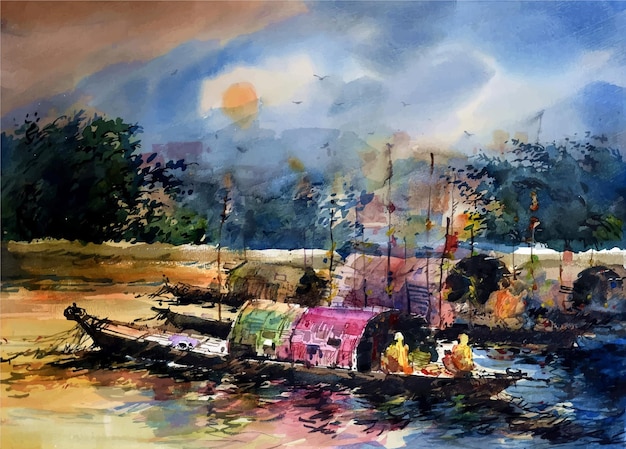This is an abstract watercolor painting characterized by its vibrant, blended colors. Dominating the scene is a brown, canoe-like boat situated in the middle, towards the bottom of the image. This boat features semi-circular roofs over its midsection, colored green and red. A smaller boat is also visible behind the main one, subtly blending into the composition. The water beneath the boats reflects a spectrum of hues: yellow on the left side, suggesting sunlight, red in the forefront echoing the roofs, and blue on the lower right. The backdrop presents a serene landscape with indistinct trees and a hint of a mountain, all rendered with soft, blurry brushstrokes typical of watercolor. The sky above is predominantly blue but transitions to orange in the upper left corner. An orangish-yellow sun is prominent in the middle of the sky, bordered by faint clouds, adding to the painting's dreamy ambiance.